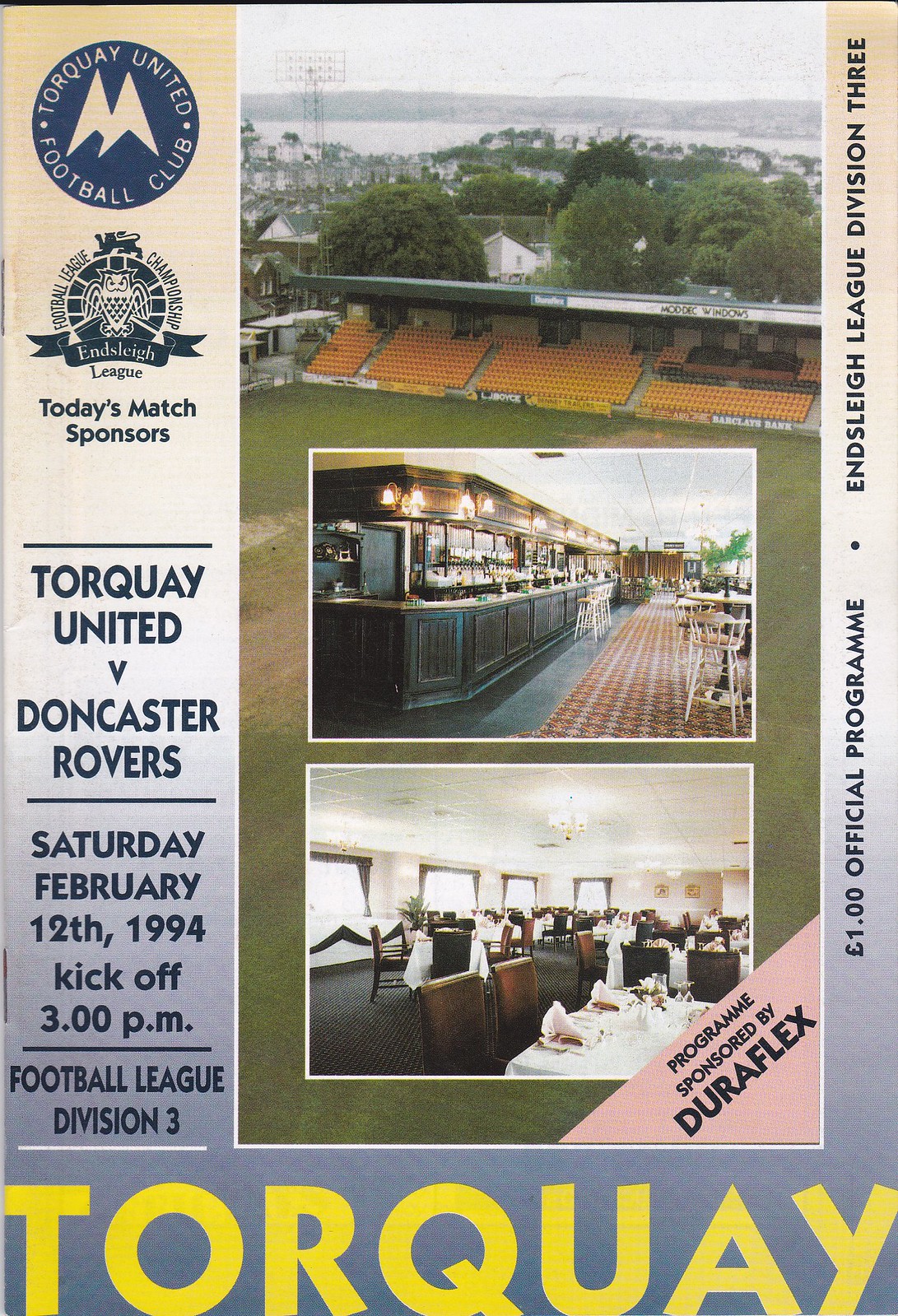The image is a vertically aligned, color-printed cover of a game day program for an event hosted by Torquay United Football Club. The program is in portrait orientation and the layout is structured in a straight vertical line. At the top left corner, there is a circular dark blue logo for Torquay United Football Club, featuring two upside-down V shapes resembling mountain peaks. Below the logo, it reads "Today's Match Sponsors" followed by the match details: "Torquay United v. Doncaster Rovers" in bold letters, "Saturday, February 12, 1994, kickoff 3 p.m." and "Football League Division III." The program cover is dominated by a large, vertical photograph of an empty football field with stadium seating in the background. Superimposed on the field are two smaller, horizontal images: the upper one depicts a bar area with seating, and the lower one shows an interior view of a dining area, both providing a glimpse of the indoor facilities. On the right side of the main photo, there is a pink corner with black text stating "Program Sponsored by Duraflex." Printed in large yellow block letters at the bottom over a blue backdrop is the word "Torquay." The right side of the cover also features a price tag, "$1 Official Program," indicating its affiliation with the Hensley League Division III.